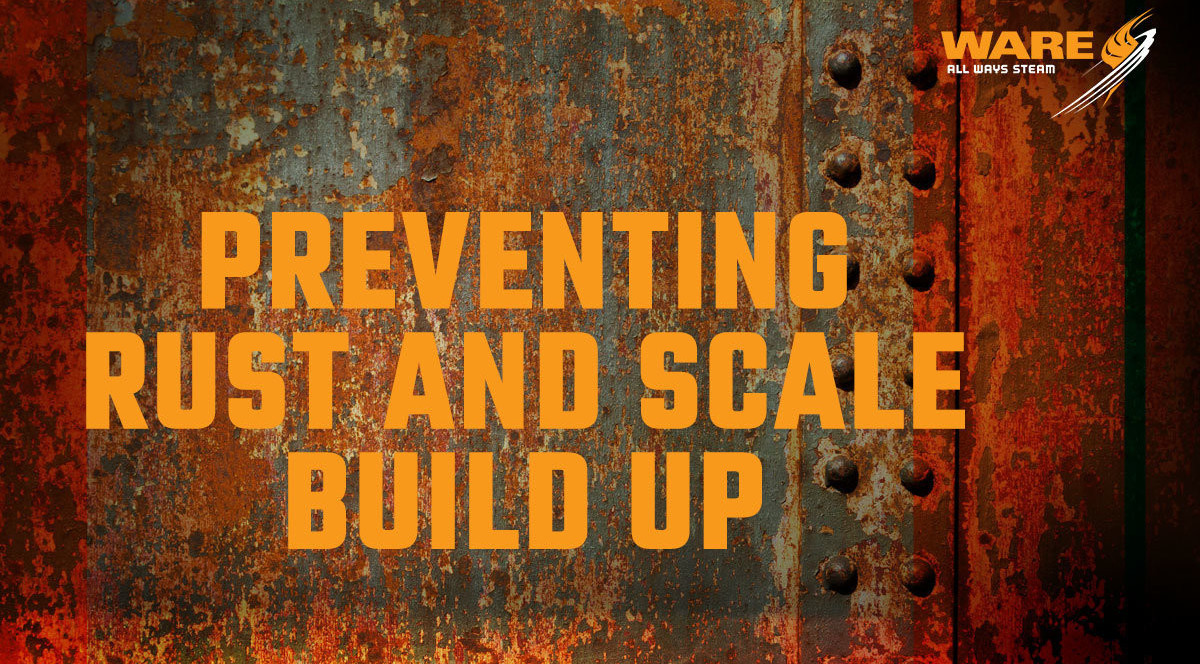This is a poster featuring a highly detailed, rusty metal background that might be from an old train car or a metal door. The metal surface is covered in heavy rust with various remnants of chipped gray and blue paint clinging to it, emphasizing its age and deterioration. Rivets and metal bracing run vertically through the metal sheet, adding to the rugged aesthetic. Over this weathered backdrop, large orange capital letters boldly state "PREVENTING RUST AND SCALE BUILD-UP." In the upper right corner, there's a logo in orange lettering spelling "W-A-R-E" followed by the slogan "always steam," accompanied by a small graphic of an orange symbol with curved white lines around it. This poster appears to be an advertisement designed to promote a product aimed at preventing rust and scale build-up, using the stark contrast of an extensively rusted metal surface to highlight the product’s necessity.